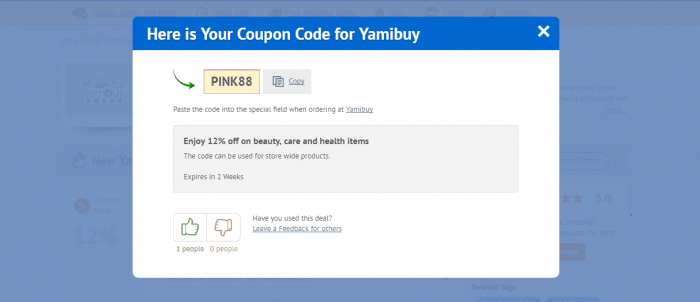Screenshot Description:

The screenshot captures a web page with a centered pop-up window containing a coupon code over a slightly blurred blue background. The pop-up has a detailed design and messaging, which appears as follows:

1. **Top Section:**
   - **Header Bar:** A blue bar at the top with white text stating, "Here is your coupon code for Yummybuy."
   - **Close Button:** An "X" in the top right corner to close the pop-up.

2. **Main Content:**
   - **Arrow and Code Box:** A green arrow points to a distinct yellow box displaying the coupon code "PINK88" in bold black letters.
   - **Instructions:** Below the yellow box, text instructions are given:
     - "Copy" next to a small icon of overlapping pages.
     - "Paste the code into the specific field when ordering at Yummybuy."
   - **Promo Details:** A text box that states, "Enjoy 12% off on beauty, care, and health items. The code can be used for store-wide products. Expires in two weeks."

3. **Bottom Section:**
   - **Feedback Area:** Icons with a thumbs up and thumbs down, labeled with "1 person" and "0 people" respectively.
   - **Feedback Prompt:** Beside the icons is the question, "Have you used this deal? Leave feedback for others."

4. **Background:**
   - Partially visible webpage elements, such as a faint ratings box in the bottom right corner and some indistinct text boxes, are obscured by the prominently displayed coupon code window.

Overall, the screenshot showcases an informative and interactive coupon pop-up designed to guide users through using the discount code on the Yummybuy website.